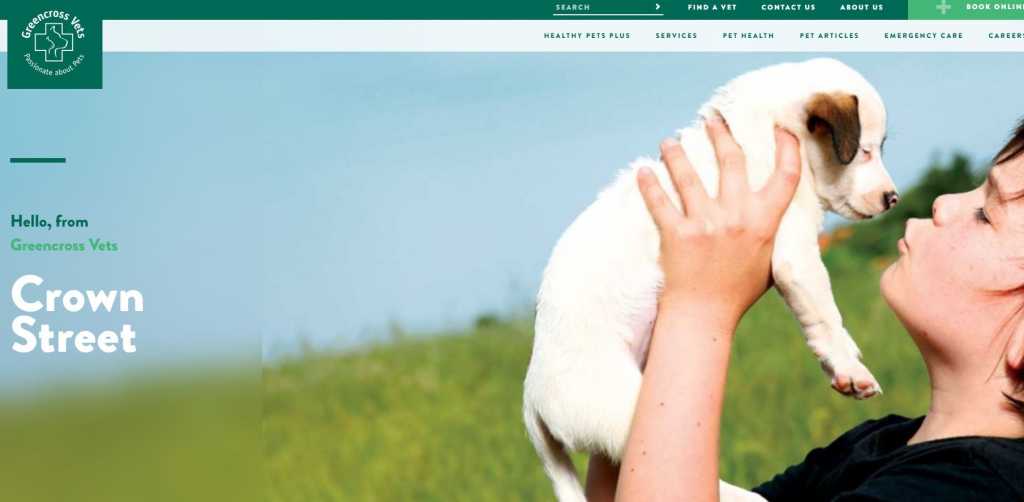The screenshot captures the homepage of a website for Green Cross Vets. At the top left corner, the website name and logo, "Green Cross Vets," are prominently displayed. Just below this header, a green line delineates the sections of the homepage. Beneath the line, the text "Hello from Green Cross Vets" is clearly visible, followed by the location name "Crown Street." On the right side of the homepage, there is a heartwarming photograph that features a child holding up an adorable small puppy. The puppy is predominantly white with distinctive brown ears, adding a charming touch to the welcoming message on the webpage.